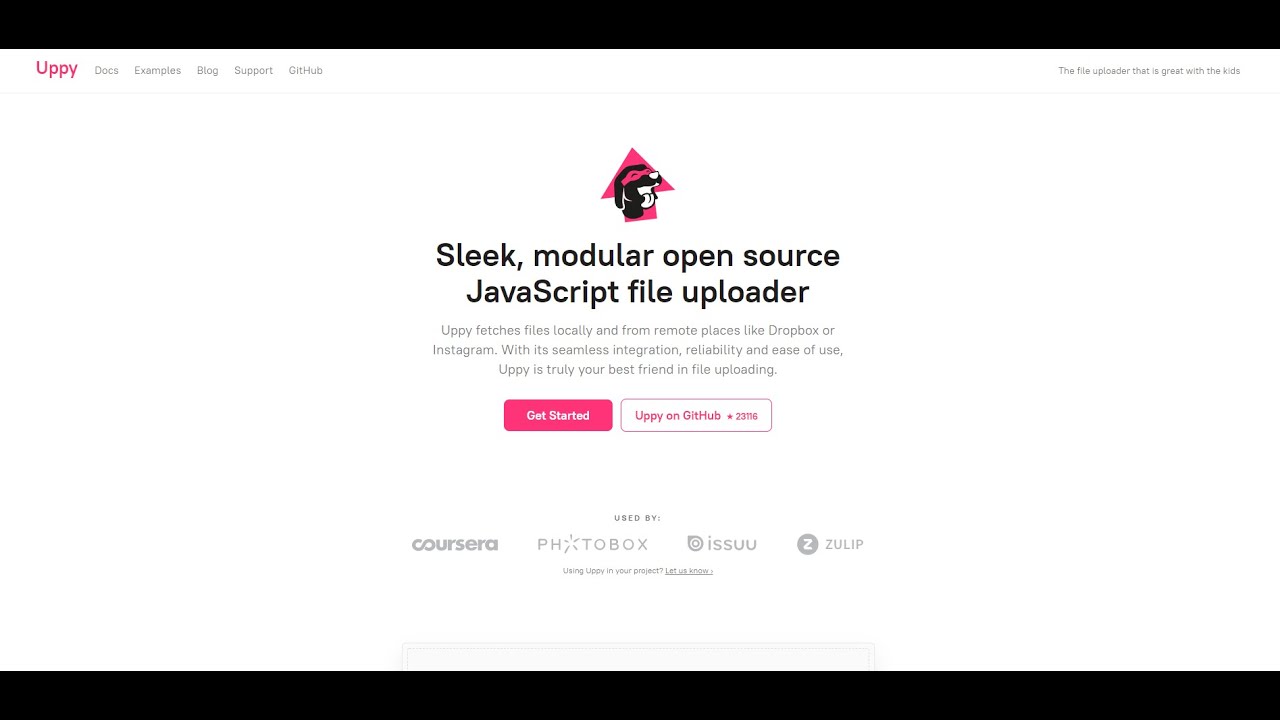The image displays a webpage for the program "Uppy." The name "Uppy" is prominently located at the top left corner in a reddish-pink color. The webpage features black borders above and below the main content area, which itself has a clean, white background. The fonts used on the webpage vary in color, ranging from the reddish-pink of the title, to light gray, and black.

To the right of the title, there are five distinct category options: "Docs," "Examples," "Blog," "Support," and "GitHub." In the far right top corner, there is a file uploader tool described as being user-friendly.

Centrally positioned on the webpage is an illustrated arrow, also in pink, featuring a black dog wearing pink goggles. The dog has a white nose and tongue and is smiling while glancing towards the right side of the screen.

Below this illustration, a headline in black font reads, "Sleek Modular Open Source JavaScript File Uploader." Further down, a paragraph in black font explains: “Uppy fetches files locally and from remote places like Dropbox or Instagram. With its seamless integration, reliability, and ease of use, Uppy is truly your best friend in file uploading.”

Two buttons are displayed below this text: a pink button labeled "Get Started" and a white button outlined in reddish-pink labeled "Uppy on GitHub *23116."

At the bottom of the page, the logos of several notable users of Uppy are shown, including Coursera, Photobox, Issuu, and Zulip. In very small font, there is a footer message that reads: "Using Uppy in Your Project? Let Us Know."